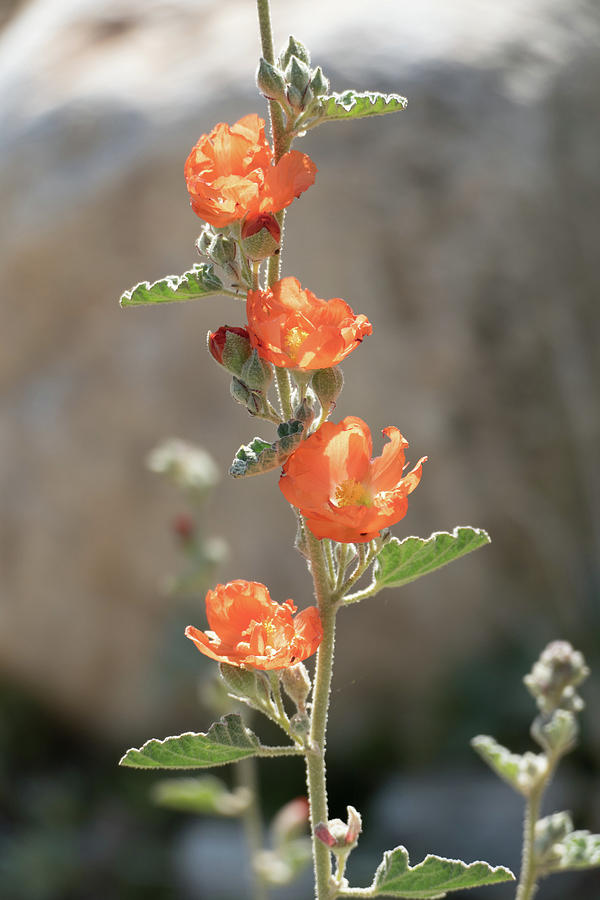This high-resolution, close-up photograph captures a slender, slightly curved plant stem extending vertically from the center-bottom to the center-top of the image, set against a blurred background that includes a light brown stone and indistinct similar plants. The subject is in sharp focus, highlighting the detailed texture and color contrasts. The stem is adorned with individual green leaves arranged alternately on each side, progressing upwards approximately half an inch apart. These leaves are small compared to the vivid orange flowers that bloom along the stem. There are four orange blossoms in various blooming stages, with the largest approximately doubling the size of the leaves. Positioned at regular intervals, each flower faces a slightly different direction—upward to the left and right. At the top of the plant, a cluster of tightly closed, green buds stands ready to bloom. Lower down, a couple of unfolding orange buds reveal hints of dark red within. The overall composition emphasizes the vibrant plant against an intentionally defocused background, ensuring that the main details of the stem, leaves, and flowers command the viewer's attention.